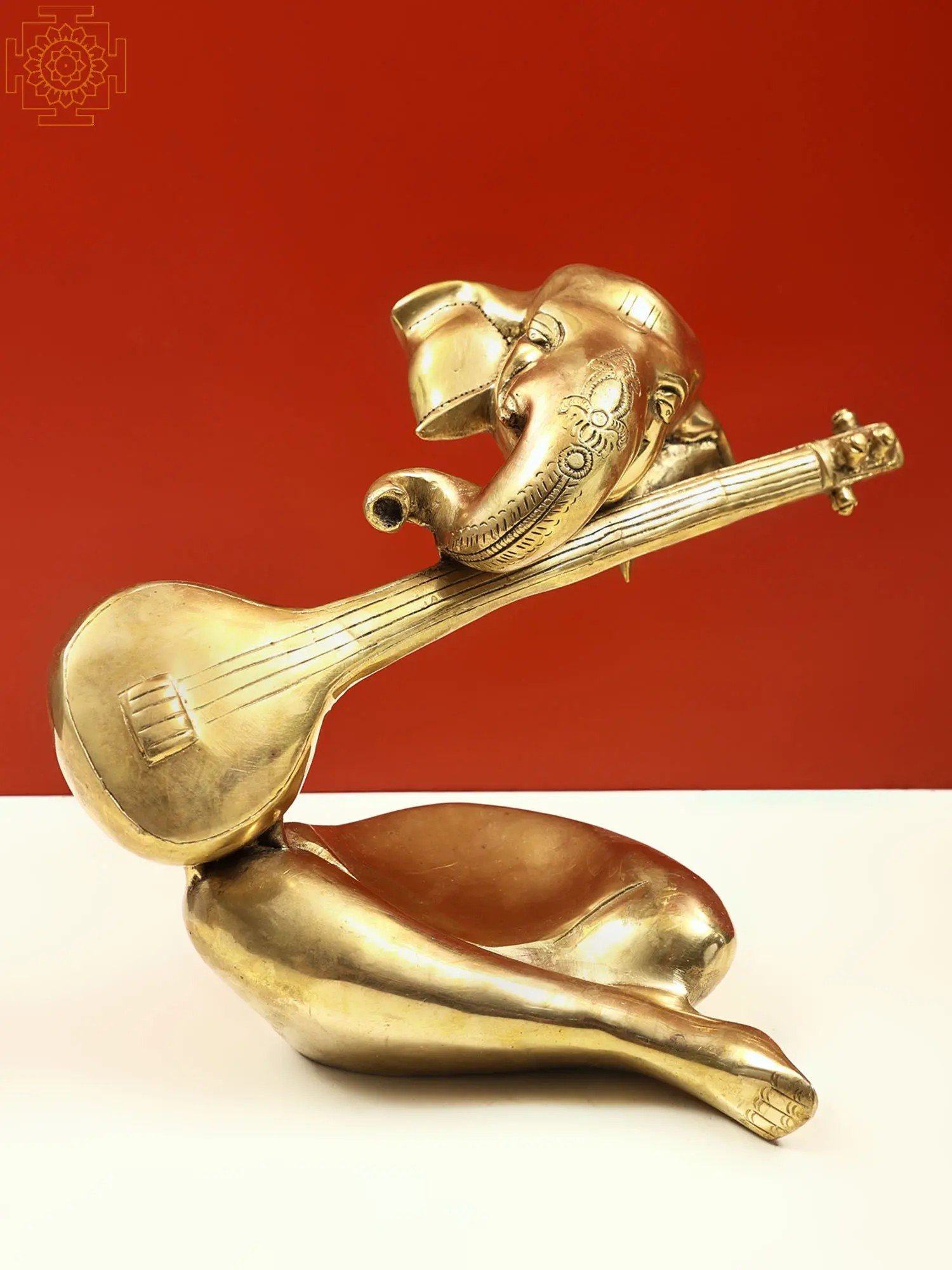A striking golden statue of the Hindu deity Ganesh is positioned on a pristine white table against a vibrant red background. This unique sculpture captures only the head adorned with intricate henna markings, part of the trunk, and the crossed legs of Ganesh. Notably, the statue is incomplete, conspicuously missing the torso, neck, and arms. In Ganesh's remaining grasp is a long-stringed instrument resembling a sitar or another traditional Indian instrument, adding to the cultural richness of the piece. The juxtaposition of the dazzling gold against the bold red and pure white further accentuates the statue’s intricate details and divine essence.